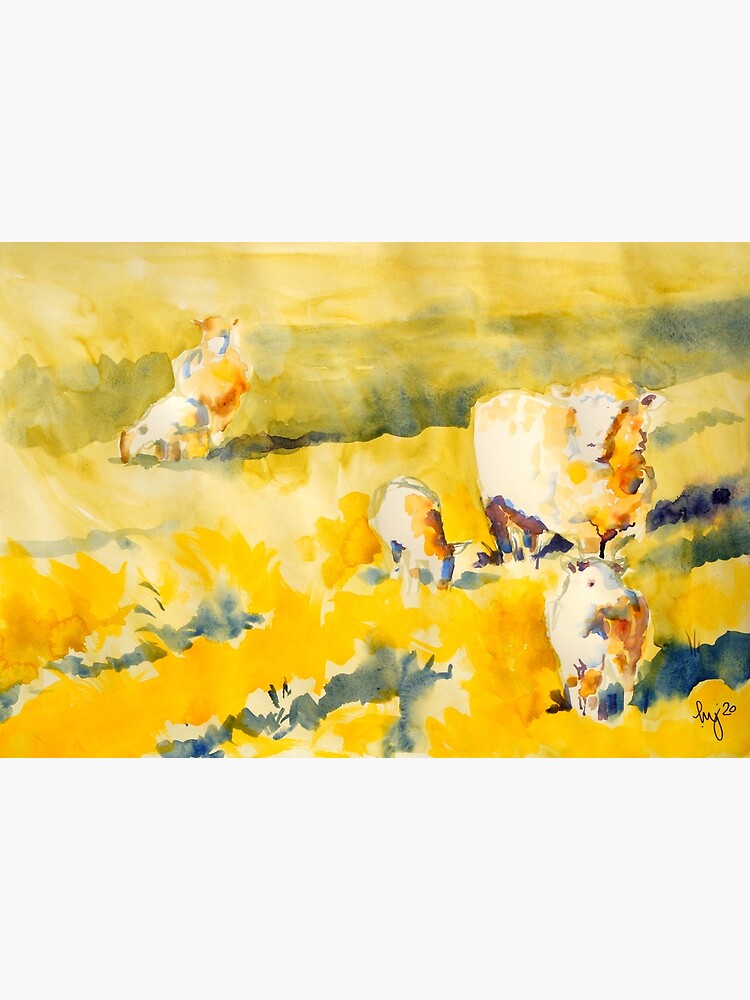The image is an abstract watercolor painting in landscape orientation, predominantly featuring varying shades of yellow and green. The scene depicts a pastoral setting where several farm animals are grazing in a field. On the right side in the foreground, there's a pig with a reddish-yellow object in its mouth, seemingly falling out. Behind the pig stands a cow, distinguishable by the cowbell around its neck, with a calf nearby to the left. Further off in the distance to the left, there's another grazing animal that appears to be another cow. Interspersed throughout the yellow field with patches of green are indistinct bluish-black elements that seem to represent bushes. Additionally, five sheep—two adult and three lambs with varying wool thickness—are also present, with the adults situated in the center facing different directions, and the lambs grazing or looking around. The golden-yellow sky and field blend together with diagonal rows of green wash cutting across the landscape. The painting is bordered by a light gray rectangle at the top and bottom, with the artist's signature reading "M-Y-X-S-20" in the lower right corner.